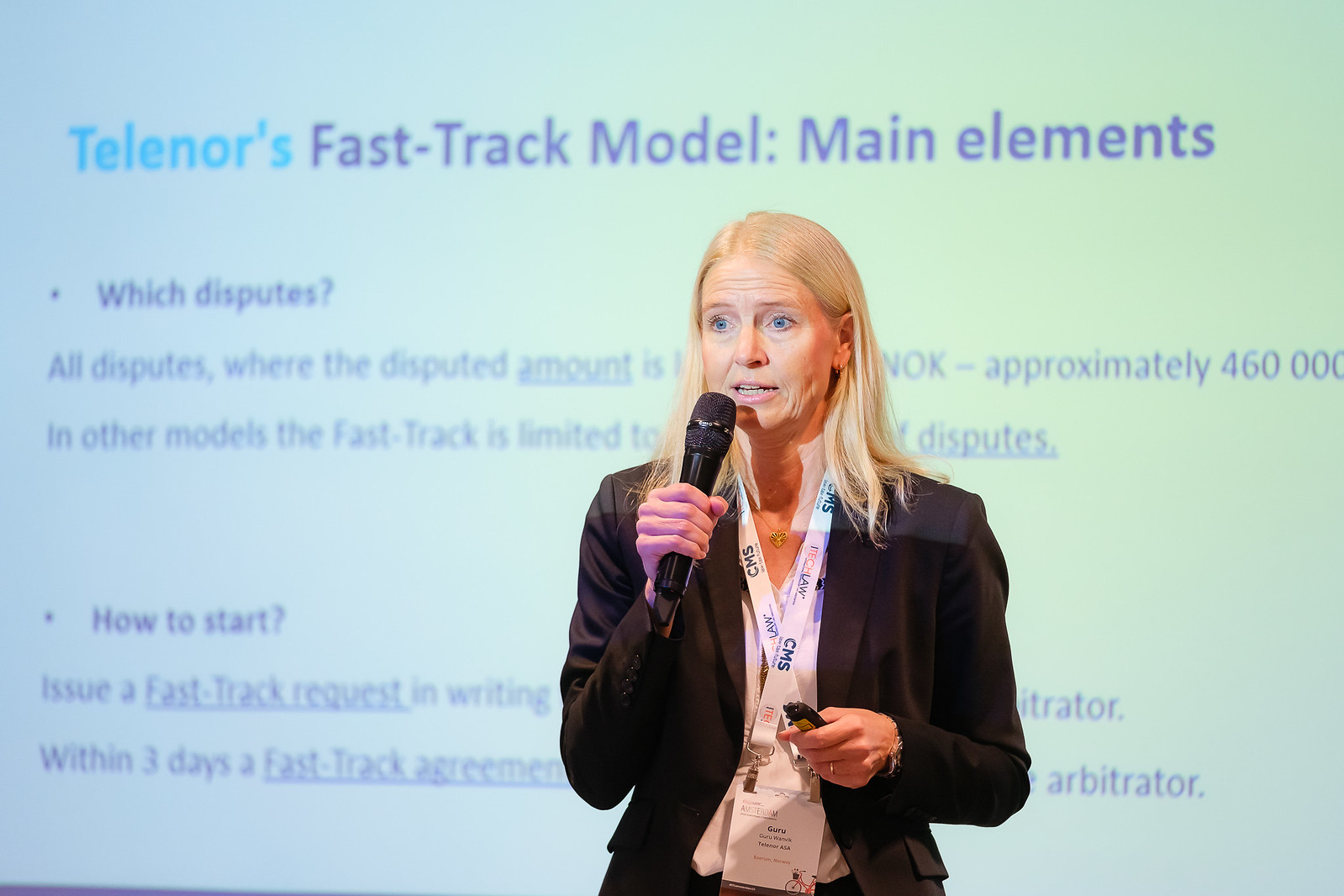A mid-aged woman with straight, blonde hair and light skin stands confidently in front of a large projection screen, which is partially obscured by her presence. She is delivering a presentation on the "Telenor's Fast Track Model: Main Elements." The visible text on the screen includes sections titled "Which Disputes?" and "How to Start." Under "Which Disputes?" it mentions "all disputes where the disputed amount is approximately $460,000," though her head partially blocks this area. Additional text hints at further details on other models but is similarly obscured. The "How to Start" section advises to issue a fast track request in writing, followed by a fast track agreement within three days. The woman, dressed in a dark jacket over a white shirt, accessorizes with a heart-shaped necklace, a lanyard bearing a name tag, and a wedding ring. She holds a black microphone close to her mouth and a clicker in the other hand, her blue eyes focused on her audience as she speaks.